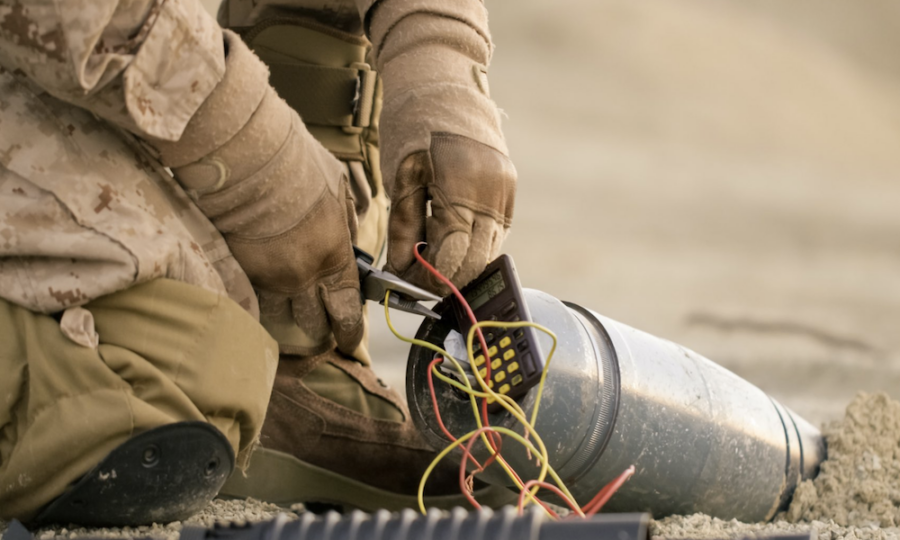The image depicts a bomb disposal expert in military attire, identifiable from the waist down, meticulously defusing an explosive device partially buried in sandy ground. Clad in brown fatigues, brown gloves, black knee pads, and green and black boots, the soldier is on one knee, deeply focused on the task at hand. His right hand wields a pair of pliers, positioned to cut a yellow wire, while his left hand steadies a red wire. These wires extend from a chrome bomb, prominently featuring what appears to be a repurposed calculator serving as a timer. The calculator, black with yellow numerals and black operational buttons, underscores the tense precision required in this high-stakes situation. Additional elements in the scene include another indistinguishable cylinder in the lower part of the frame, hinting at the complexity and danger faced by the bomb defusal expert.